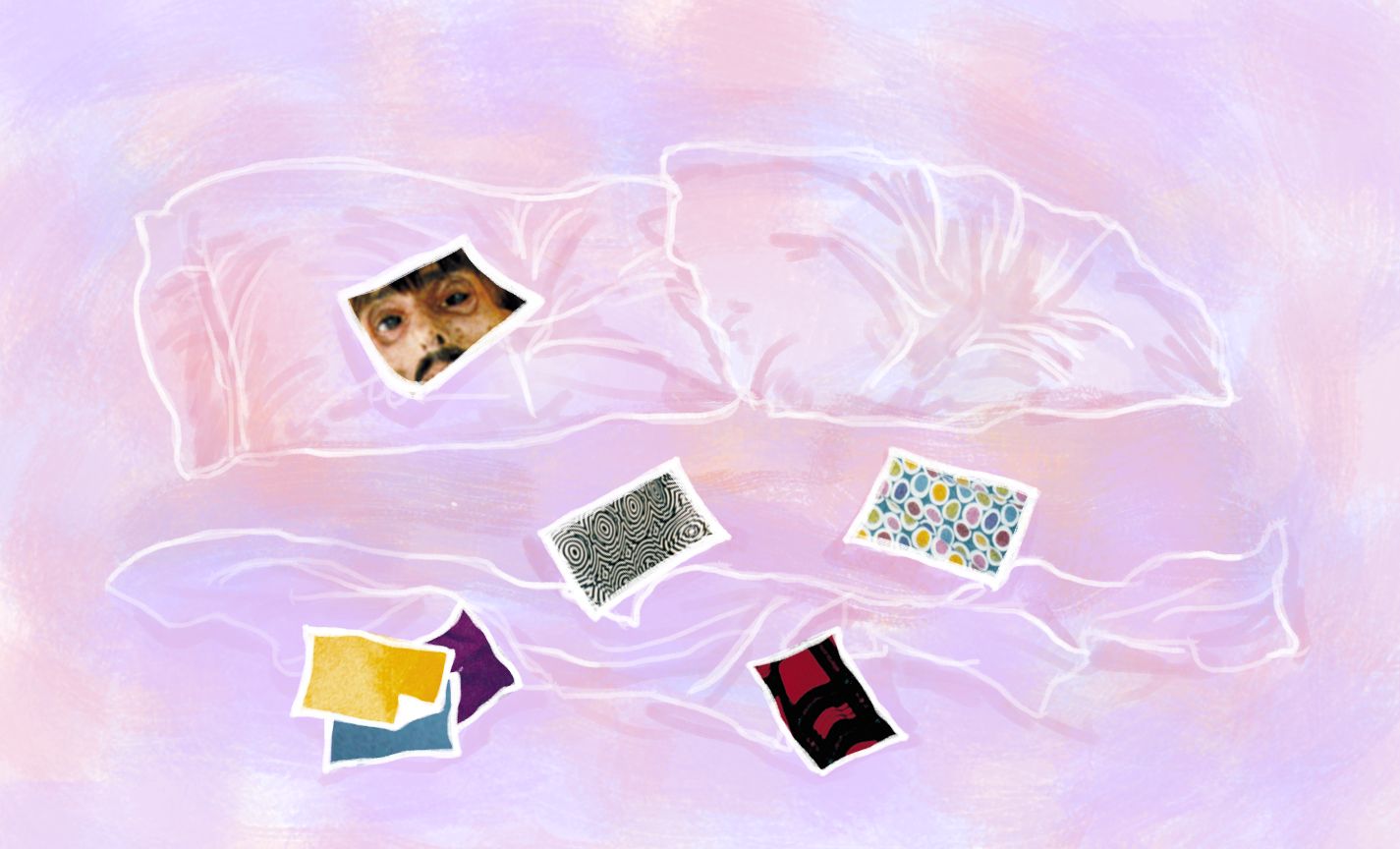The image depicts an abstract artwork with a pastel-colored background, featuring a mixture of pinks, whites, purples, and light blues gently blending into each other, creating a soft and subtle texture. Over this pastel backdrop, there are white chalk-like outlines resembling crumpled paper or loosely sketched elements, forming two pillow shapes and a bedspread. On this textured canvas, several distinct and abstract images are superimposed, each bordered by a thick white frame, reminiscent of postcard-sized photographs or fabric samples. In the bottom left corner, there are three solid blocks of color in gold, blue, and purple. Among the various images, one prominently features a close-up of a man's face with black hair and a mustache. Other images include a paisley pattern, polka dots, and a piece of cloth with red and black stripes. The composition lacks signatures or distinctive marks from the artist, adding to its enigmatic charm.